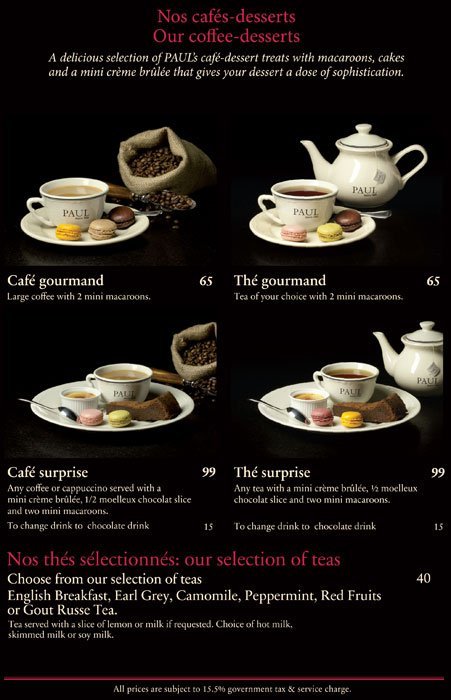The image depicts a stylish black magazine advertisement featuring a series of tea sets arranged in a vertical, rectangular format. At the top, the text reads "Nos Cafe Desserts, Our Coffee Desserts: A delicious selection of Paul's Cafe Dessert Treats with macarons, cakes, and a mini crème brulee that gives your dessert a dose of sophistication." The four options are organized in a two-by-two grid, each showcasing different dessert and beverage combinations.

1. **Cafe Gourmand**: A large coffee served with two mini macarons, priced at 65.
2. **Tea Gourmand**: Tea of your choice with two mini macarons, priced at 65.
3. **Cafe Surprise**: Any coffee or cappuccino with a mini crème brulee, half a slice of Moyes chocolate cake, and two mini macarons. Optionally, you can switch the drink to hot chocolate for an additional 15, with a total price of 99.
4. **Tea Surprise**: Any tea with a mini crème brulee, half a slice of Moyes chocolate cake, and two mini macarons. Switching the drink to hot chocolate also costs an additional 15.

Towards the bottom, there's a selection of teas listed: English Breakfast, Earl Grey, Chamomile, Peppermint, Red Fruits, and Gout Roast Tea, priced at 40. Smaller text elaborates that tea is served with a slice of lemon milk if requested, with choices of milk including soy milk and skim milk. The advertisement features a sophisticated, visually appealing design aimed at highlighting the elegance and variety of Paul's Cafe dessert offerings.